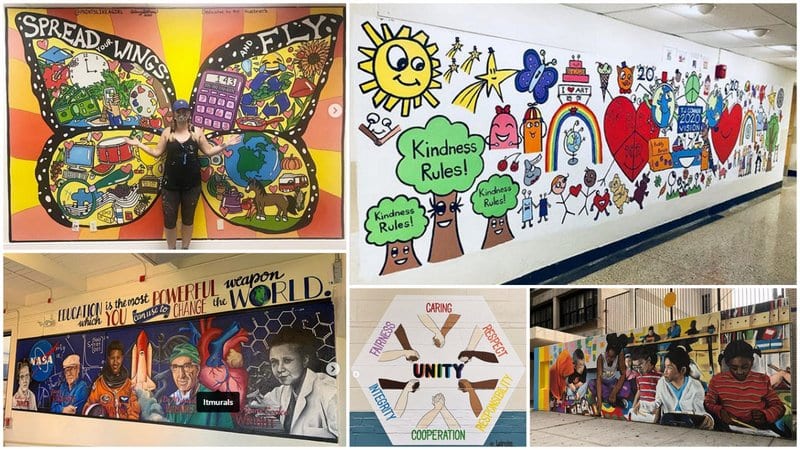This captivating photograph displays a collage of five distinct murals commonly seen in a school setting. The top left image features a woman posing in front of a vibrant butterfly mural with the inspirational phrase "Spread Your Wings and Fly." Each butterfly wing segment is filled with diverse symbols, including clocks, calculators, globes, emojis, magnifying glasses, and various other shapes. The top right image, the largest in the collage, showcases a colorful mural along a well-lit school hallway. It depicts trees with the phrase "Kindness Rules," accompanied by sunshine, hearts, butterflies, and stick figure children playing. The bottom left image highlights influential figures in history with a NASA theme, including astronauts, space shuttles, and renowned scientists. The bottom middle mural promotes unity through an illustration of intertwined hands of different colors, representing fitness, caring, respect, responsibility, cooperation, and integrity. Lastly, the bottom right image shows a mural of a classroom scene with children, likely around seven years old, sitting in a circle on the floor, engaged in reading. Each mural offers motivational messages and vibrant artwork, enhancing the school’s educational and inspirational environment.